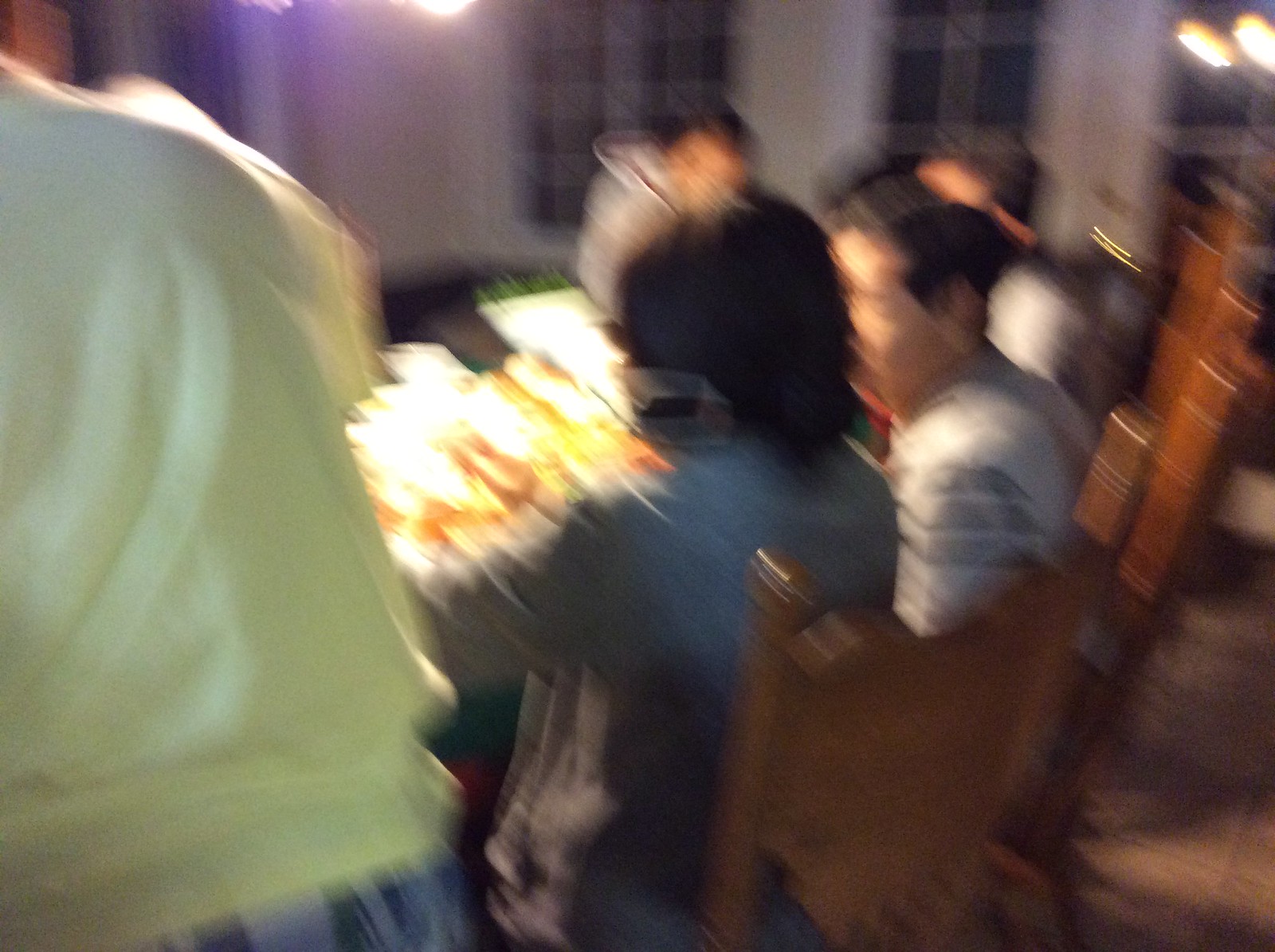A blurred photograph captures a warm family gathering around a large, oval-shaped dining room table. Despite the indistinct outlines, the high-backed chairs made of rich, dark brown wood are distinguishable. A person is seen standing, possibly delivering a tray to the table or preparing to sit. Two other individuals are seated, engaging in what appears to be a shared moment. The table itself reflects a bright light source, hinting at the glassware or polished surface. Above, the soft glow of a chandelier's bulb adds a touch of elegance to the cozy scene.